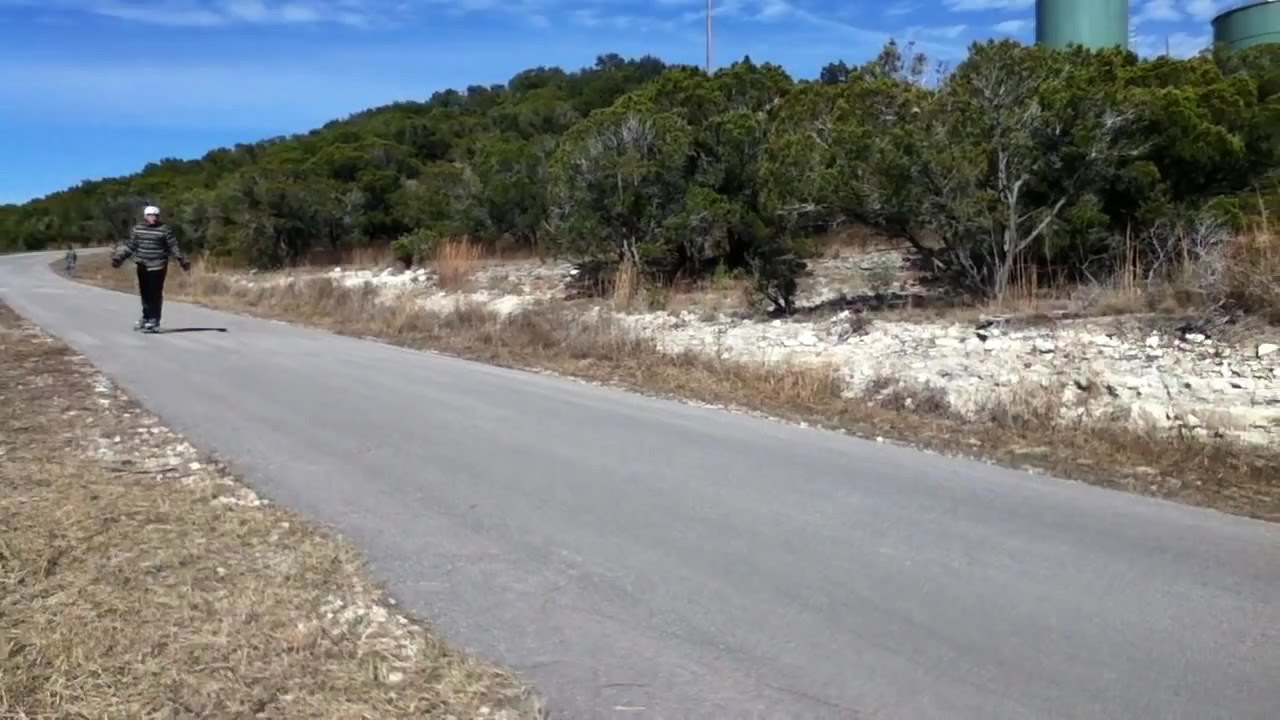In the photograph of a desert scrubby area, a solitary blacktop road runs down the center, devoid of any vehicles. The terrain on either side of the road features low, sparse grasses interspersed with white rocks. To the right, a cluster of low green trees lines the roadside, alongside patches of brownish and whitish land, possibly showing sand or light snow. Standing still in the middle of the road, a person, presumably a man, faces the camera with arms slightly outstretched, clad in black pants and a black and white striped shirt, and wearing a white helmet. The clear blue sky with a few white clouds indicates a sunny day. In the backdrop on the right side, there are two green cylindrical structures, resembling either tanks or factory silos, adding an industrial touch to the otherwise natural landscape. A figure further back along the road is faintly visible, hinting at a possibility of someone skateboarding or roller-skating towards the viewer.